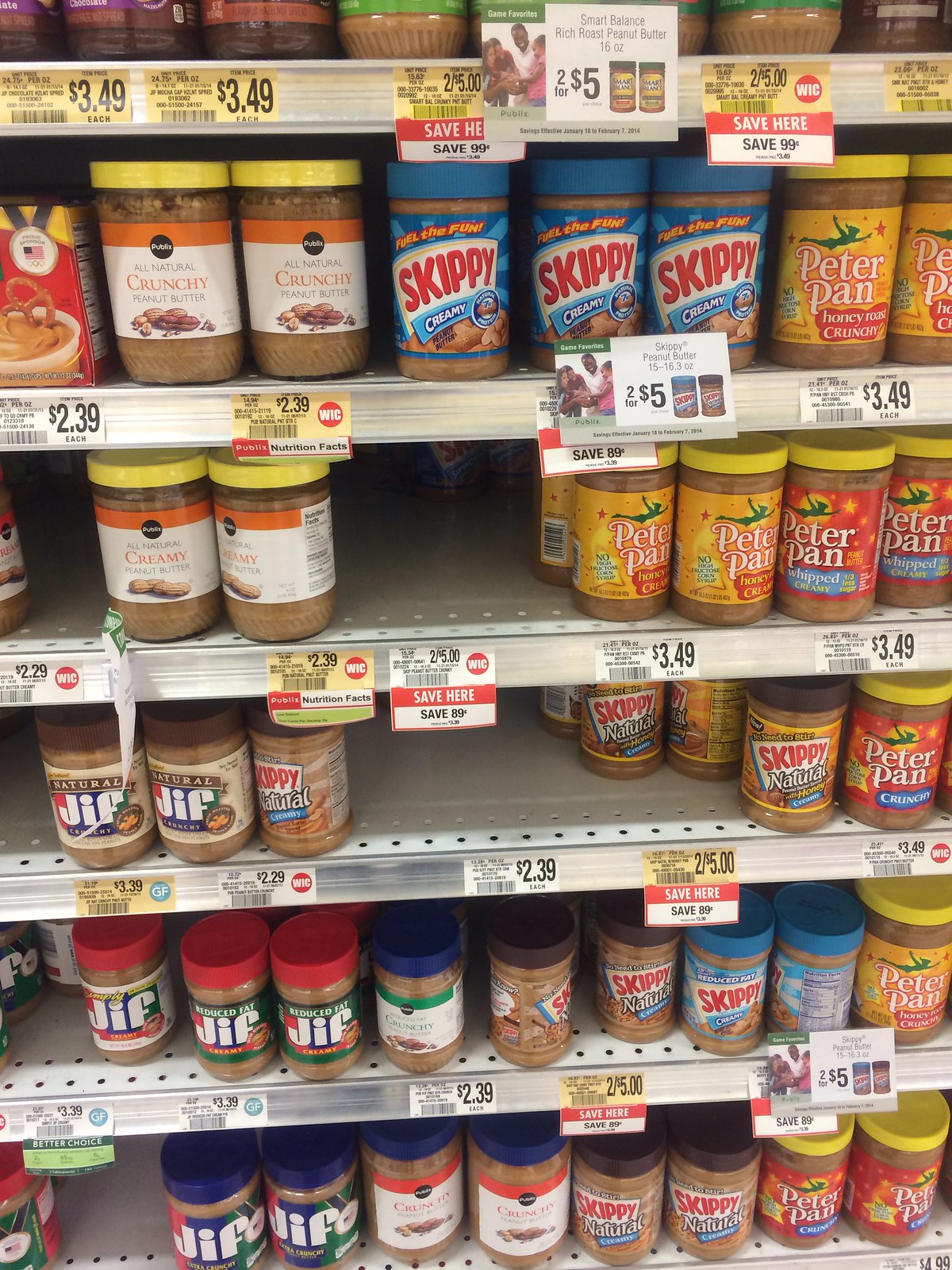This photograph showcases the peanut butter section of a supermarket aisle, featuring approximately six shelves filled with various brands and types of peanut butter. On the top shelf, there are cans of crunchy peanut butter from an off-brand, natural variety. Adjacent to these are jars of creamy Skippy in blue containers, followed by honey and crunchy Peter Pan in their characteristic yellow jars with a red label.

The second shelf displays the same off-brand natural peanut butter, but in a creamy variety. This shelf also includes an empty spot where a type of peanut butter is sold out. Next to the empty spot, there are honey, creamy, and whipped creamy Peter Pan jars.

The third shelf houses jars of Jif, natural Skippy, and Peter Pan crunchy varieties. The detailed labels feature blue lids with red lettering for Skippy, yellow lids with a mix of red and yellow on Peter Pan jars, and the unmistakable branding of Jif.

Prices for these items range from $2.29 to $3.49, as indicated on the shelf tags below each item, many of which include savings offers. The shelves themselves are standard supermarket issue with steel or aluminum front pieces that hold the price tags, and baked enamel metal shelving with perforation lines running down the edges for added stability.

Overall, the variety is dominated by major brands like Jif, Skippy, and Peter Pan, interspersed with off-brand natural options, catering to a wide range of peanut butter preferences.